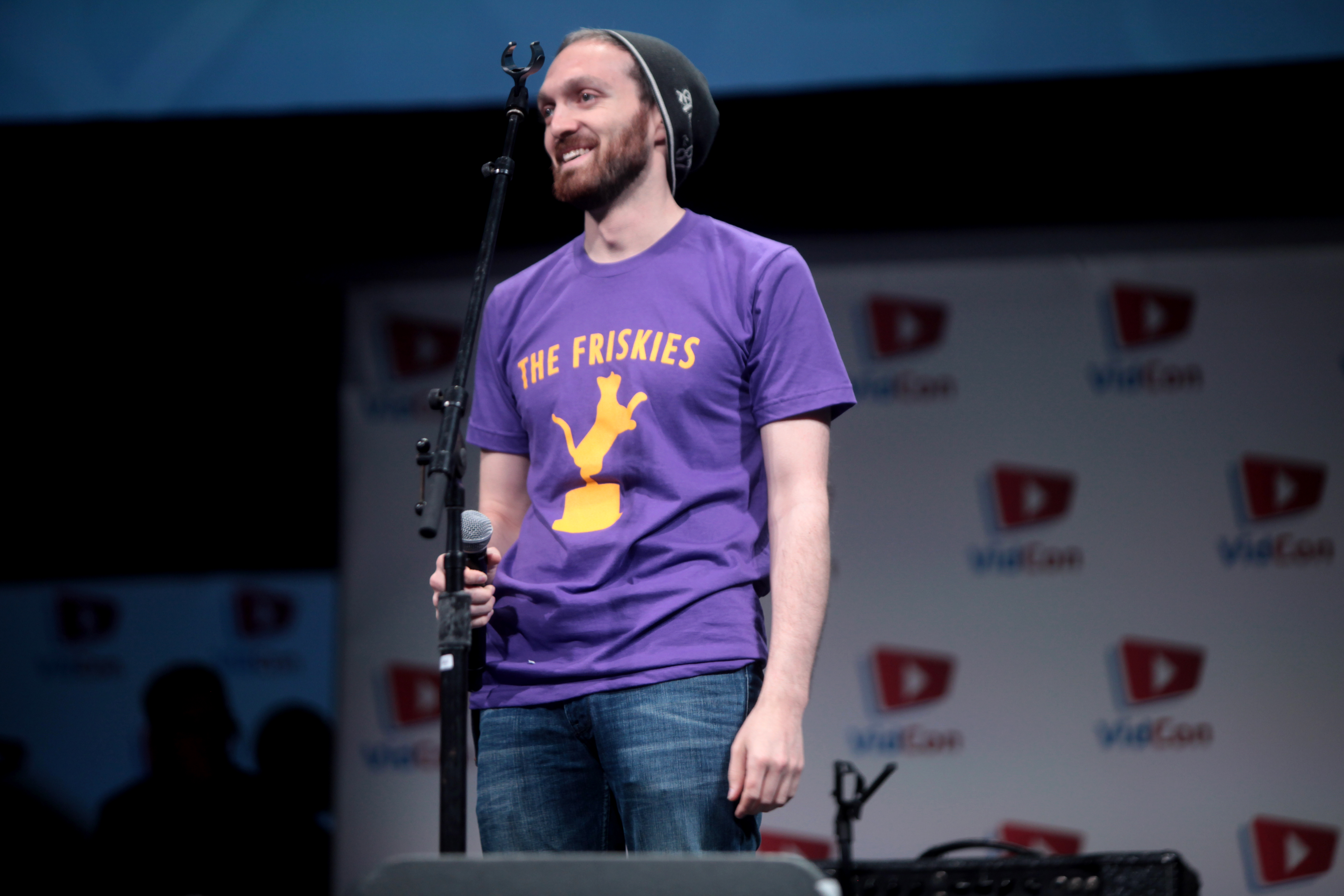In this photo, a young Caucasian man is standing on a stage, presumably at an event like VidCon, judging by the blurred backdrop that seems to indicate such. He appears to be engaged in a presentation or a Q&A session, evidenced by the microphone he holds in his right hand and the empty microphone stand positioned in front of him. The microphone has a black base with a silver head. The man is smiling and looking slightly off-camera to the left, giving the impression of interacting with his audience. He is wearing a dark-colored slouch beanie with a light gray lining, which covers most of his dark brown hair. His facial features include a reddish-brown beard and brown eyes. He is dressed in a purple short-sleeve t-shirt with orange lettering that reads "The Friskies," featuring a silhouette of a cat standing on a box. He pairs this with medium blue jeans. An amplifier is visible at the front of the stage, and the overall setting suggests a professional event, even though he is not looking directly into the camera.